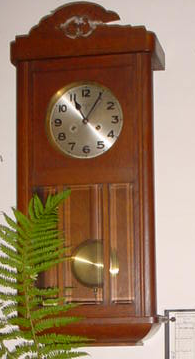The image captures a detailed close-up of a small, old-fashioned grandfather clock hanging on an off-white wall. The clock, made of rich chocolate brown wood, showcases intricate carvings at its top, possibly resembling birds or cloud-like shapes. The clock face is a striking metallic silver, surrounded by an elegant gold border. The numbers and hands on the face are black, with the hour hand pointing to 11 and the minute hand at 1. Two small white-centered circles on the clock face indicate wind-up points. 

A prominent gold pendulum is visible through a rectangular glass panel at the bottom of the clock, adding to its vintage charm. To the left, a dark green fern branch partially obscures the lower part of the clock. In the background, the right side of the frame hints at another piece of decor—a picture frame with indistinguishable drawing lines and a black border. The composition is vertical, emphasizing the clock's elongated form and the wall's off-white hue.